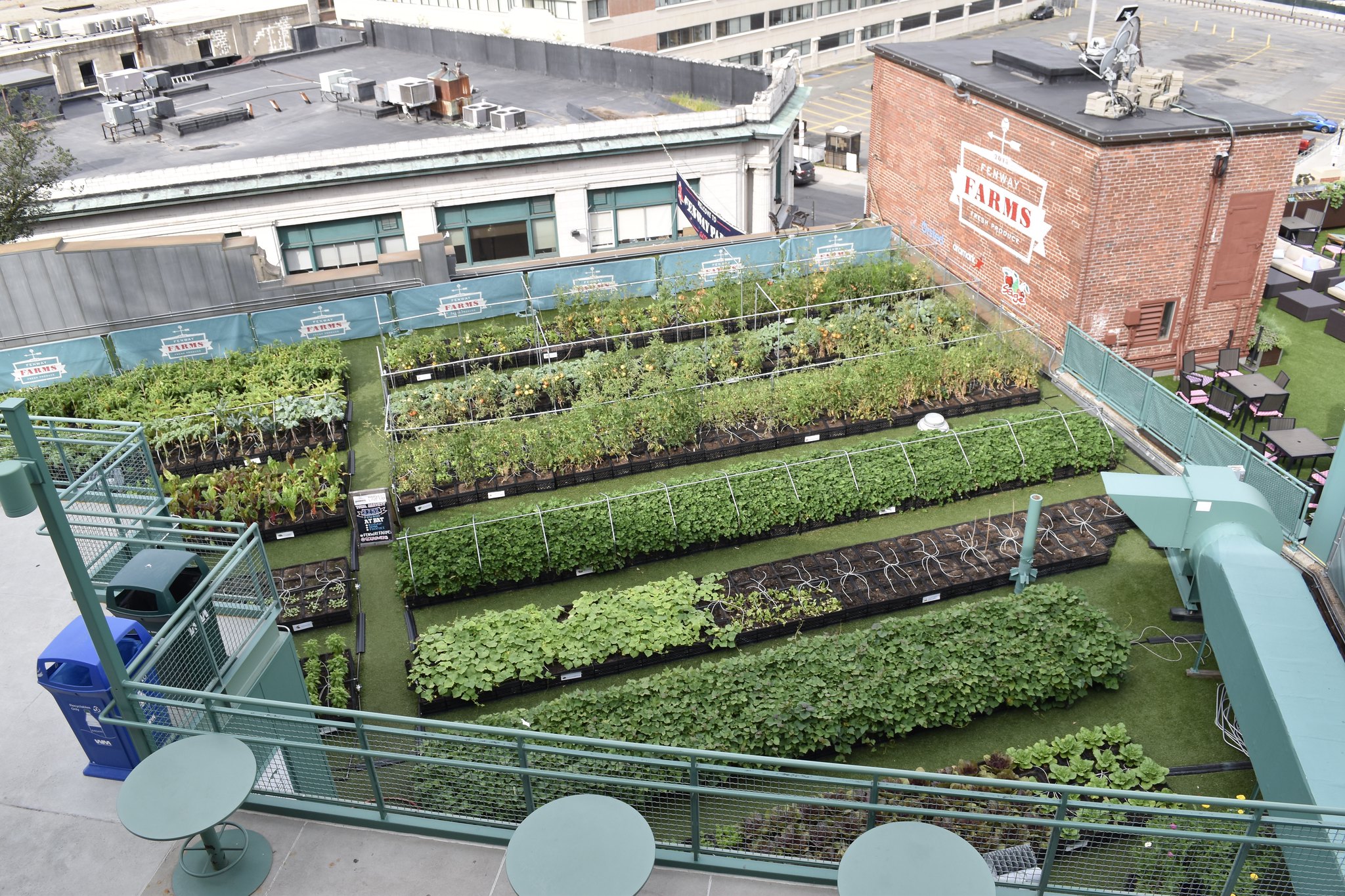This captivating overhead color photograph features a meticulously maintained rooftop garden, prominently showcasing the vibrant urban oasis known as Fenway Farms. Situated on a reddish-orange brick elevator shaft or industrial section of the rooftop, the Fenway Farms name, accompanied by a wind vane logo, is clearly visible. The garden itself is surrounded by a green fabric fence adorned with additional logos of Fenway Farms, providing wind protection.

In the foreground, an elevated patio or balcony area offers an inviting space with black tables, patio chairs, and couches, all set on green astroturf. Nearby, there are disposal areas for litter and recyclables, including blue and green recycling bins. The garden is lined with rows of crops in raised containers, with some featuring metal trellises above them and drip irrigation systems in place to ensure the plants thrive.

Adjacent rooftops house air conditioning units and satellite dishes, adding to the urban ambiance. Beyond the garden, we see several more tables and chairs on another rooftop section, blending seamlessly into the urban landscape that includes office buildings and parking lots in the background. This beautifully maintained rooftop garden exemplifies a perfect blend of urban agriculture and community space.